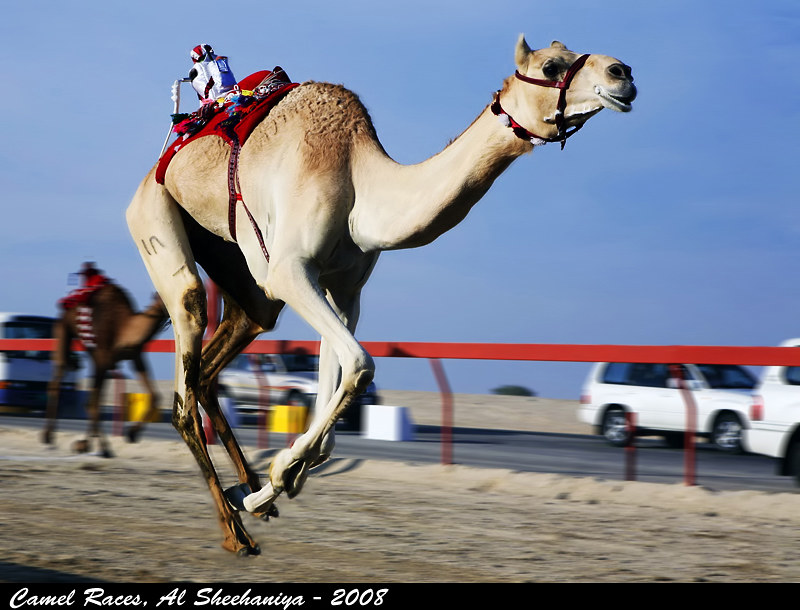This rectangular color photograph, wider than it is tall, features a vivid scene from the "Camel Races, Al-Shihanya 2008," as indicated by the white lettering on the black border at the bottom of the image. Dominating the foreground, a pale camel, adorned with a decorative red saddle blanket, hurtles forward against the dirt track, its front legs notably lighter than its brown back legs. Strapped around its face and neck, the camel wears gear, and it appears to be smiling as it races. The background reveals another camel, darker brown and slightly blurred, similarly equipped and also running. Both camels are separated from a road by a striking red barrier that spans the width of the photo. Beyond this boundary, a clear blue sky overlooks a road with several vehicles, including white, boxy SUVs and sedans, some blurred by motion. The overall composition creates a dynamic snapshot of the racing event, capturing the energy and excitement of the moment.